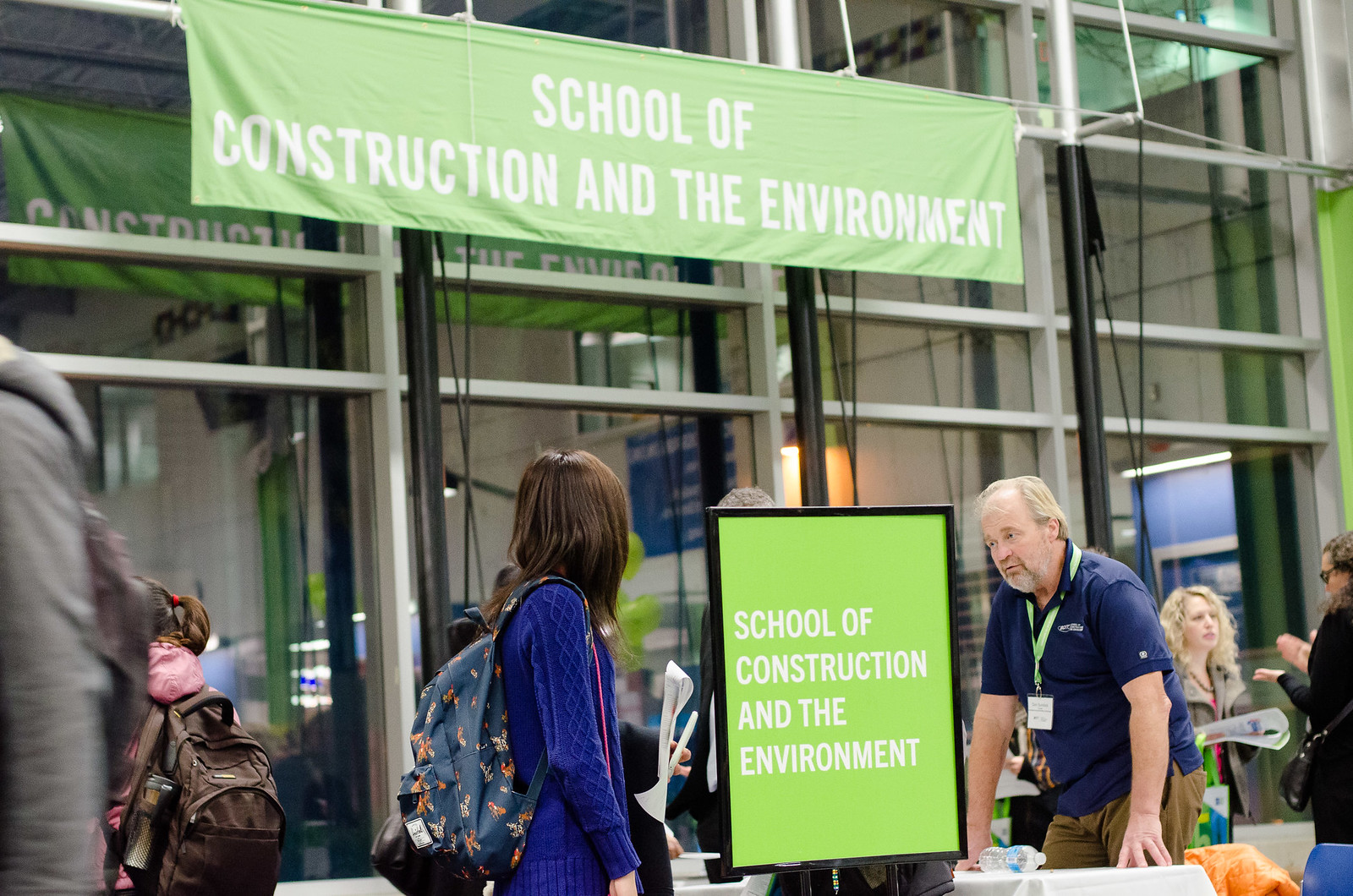In this image, you see a bustling outdoor setting, possibly at a convention or fair, dominated by a green banner that reads "School of Construction and the Environment" in white letters. The banner is prominently displayed on a steel scaffolding structure with grey metal bars running vertically and horizontally. At ground level, there is a green sign with the same text in white, encased in a black frame. 

In the foreground, an older, balding man with white hair is visible. He is wearing a blue short-sleeve shirt and brown trousers, with a lanyard and badge around his neck, indicating he is likely part of the event staff. He appears to be engaging in conversation with a woman who has long brown hair and is dressed in a blue sweater and a backpack adorned with a pattern, possibly butterflies or fish. Her back is turned to the camera, and she is holding papers as she interacts with the man.

In the background, several people are either walking by or standing and talking, some carrying papers and wearing backpacks, adding to the lively atmosphere of the scene.